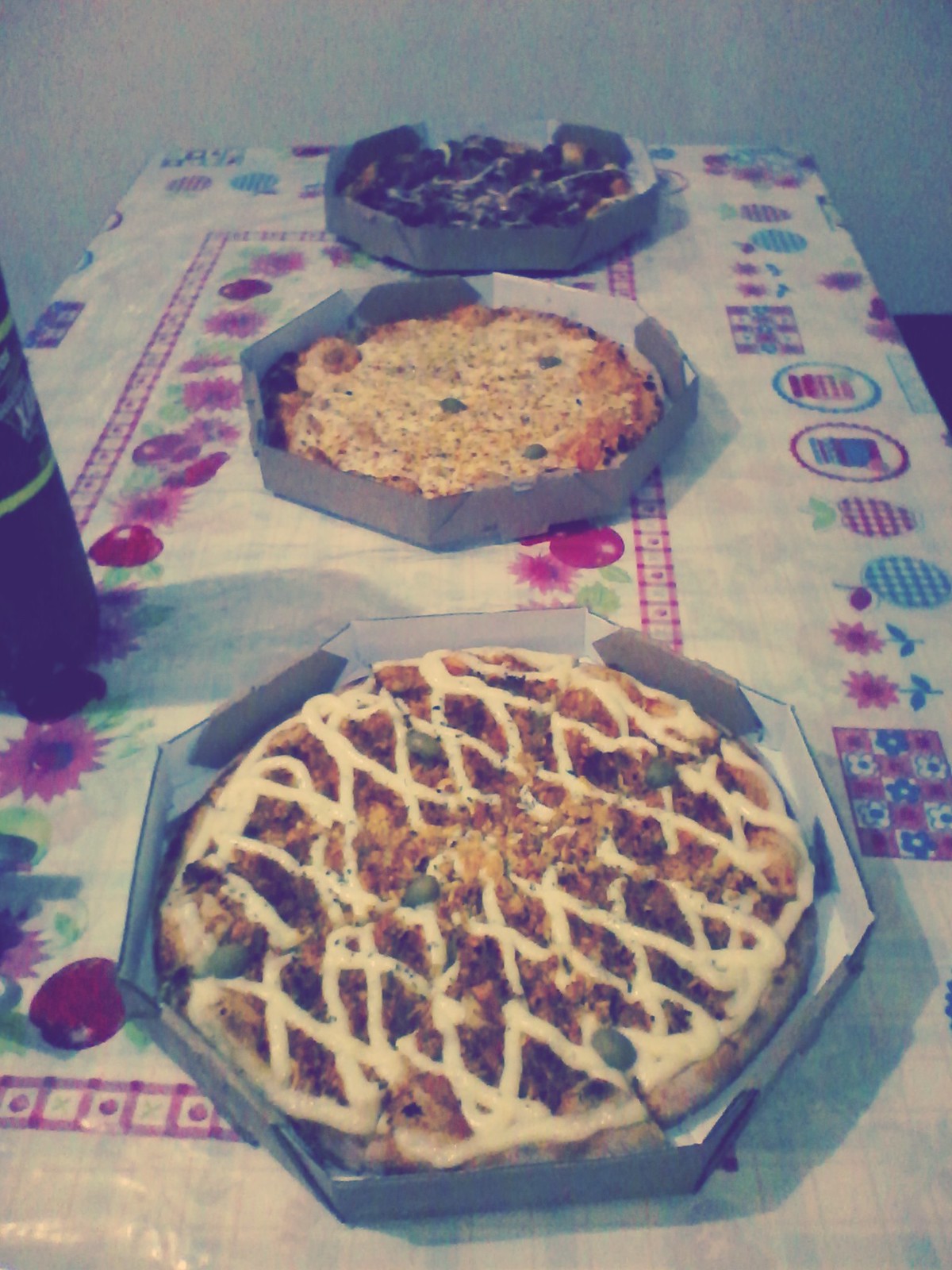A colorful and busy picnic table is adorned with a multicolored tablecloth featuring an old-fashioned checkerboard pattern interspersed with images of fruits and flowers in blues, pinks, purples, reds, and greens. Atop the tablecloth, a wine bottle with a distinctive yellow, white, and black label stands near the center. The table boasts an enticing display of three desserts, each housed in octagonal paper holders. The dessert on the left resembles an apple crisp with a dollop of white cream on top, while the middle dessert appears to be a cheese Danish or perhaps a cheese pizza, and the third dessert on the right seems to include chocolate, with a dark-colored filling. There is a rustic charm, enhanced by a small bench positioned to the right of the table. The setup suggests a delightful outdoor dining experience.